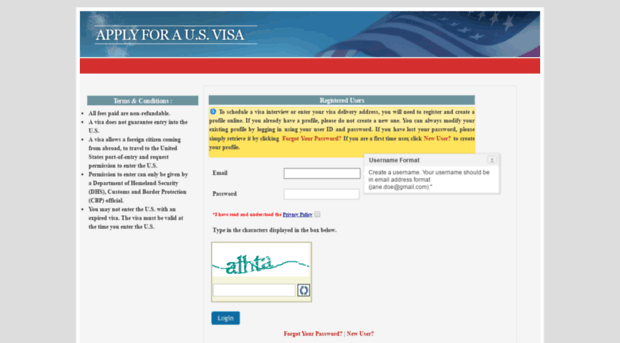The image appears to be a screenshot of a website for applying for a U.S. Visa. At the top left corner of the website, there is a header that reads "Apply for a U.S. Visa," accentuated by white horizontal lines both above and below the text. In the background to the right of this text, the American flag is depicted billowing in the wind against a backdrop of a blue sky.

Towards the middle left side of the image, the section titled "Terms and Conditions" is visible. Under this section, five bullet points are listed:
1. All fees are non-refundable.
2. A visa does not guarantee entry to the U.S.

On the right-hand side of the "Terms and Conditions" section, there is a "Registered Users" section, featuring a login form. This form includes fields for "E-mail" and "Password," each accompanied by corresponding input boxes.

At the bottom middle of the image, there is a CAPTCHA verification box for user authentication. The CAPTCHA challenge requires users to type the characters displayed in the image, which spells out "ALHTA."